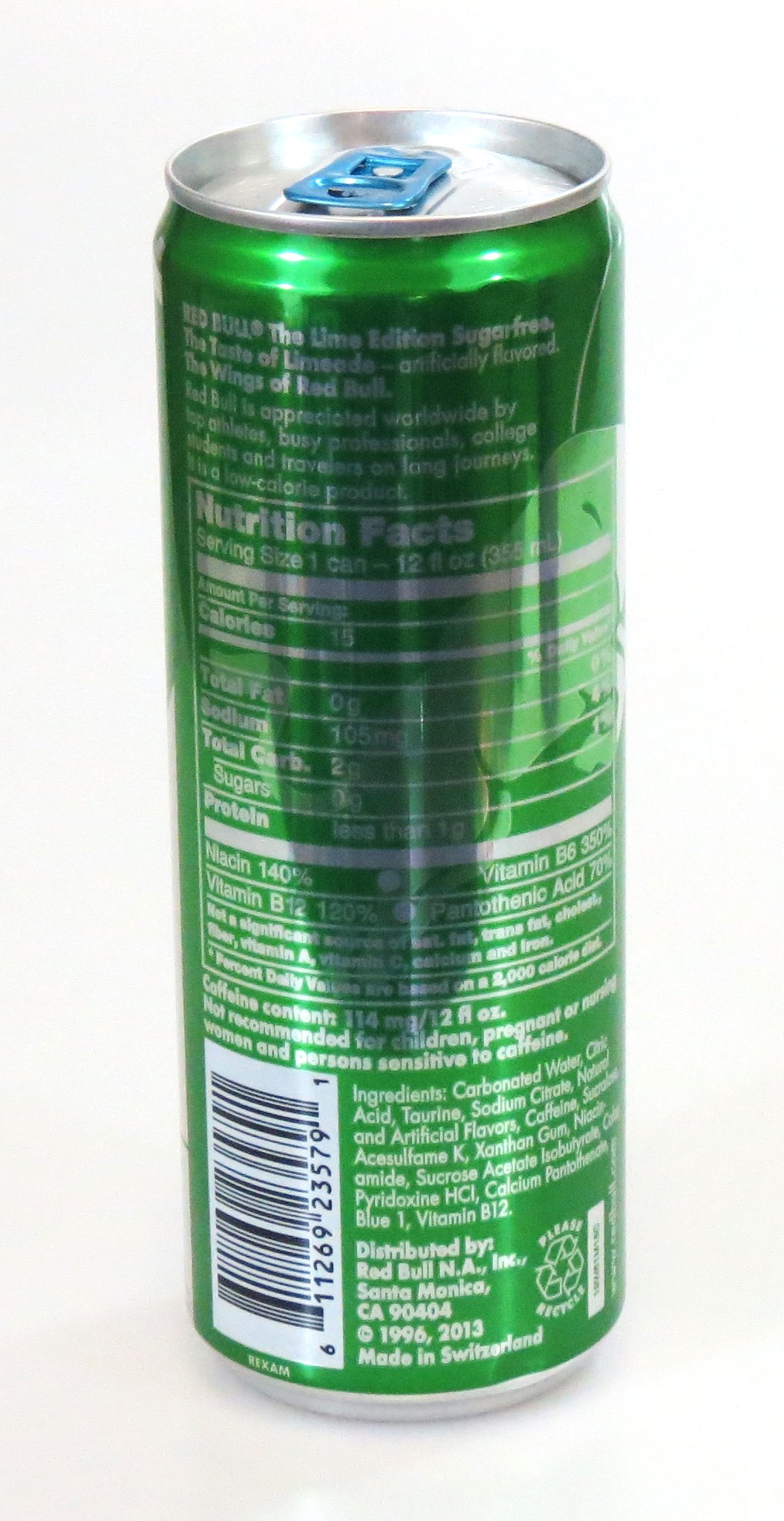A vivid green can of Red Bull's Lime Edition, a sugar-free energy drink, prominently displays its signature logo "Red Bull gives you wings." The can describes the beverage as having the refreshing taste of artificially flavored lemonade. It boasts a range of nutritional information: a single can is 15 calories with zero fat, 105 milligrams of sodium, 2 grams of carbohydrates, and less than a gram of protein. It provides 140% of the daily value for niacin and 120% for vitamin B12, while packing 314 milligrams of caffeine in each 12-ounce serving. The drink is not recommended for children, pregnant or nursing women, and individuals sensitive to caffeine. Its ingredients include carbonated water, citric acid, taurine, sodium bicarbonate, artificial flavors, caffeine, acesulfame potassium, and xanthan gum. Distributed by Red Bull North America, Inc., based in Santa Monica, California, the product is made in Switzerland and has been part of their lineup since 2013.